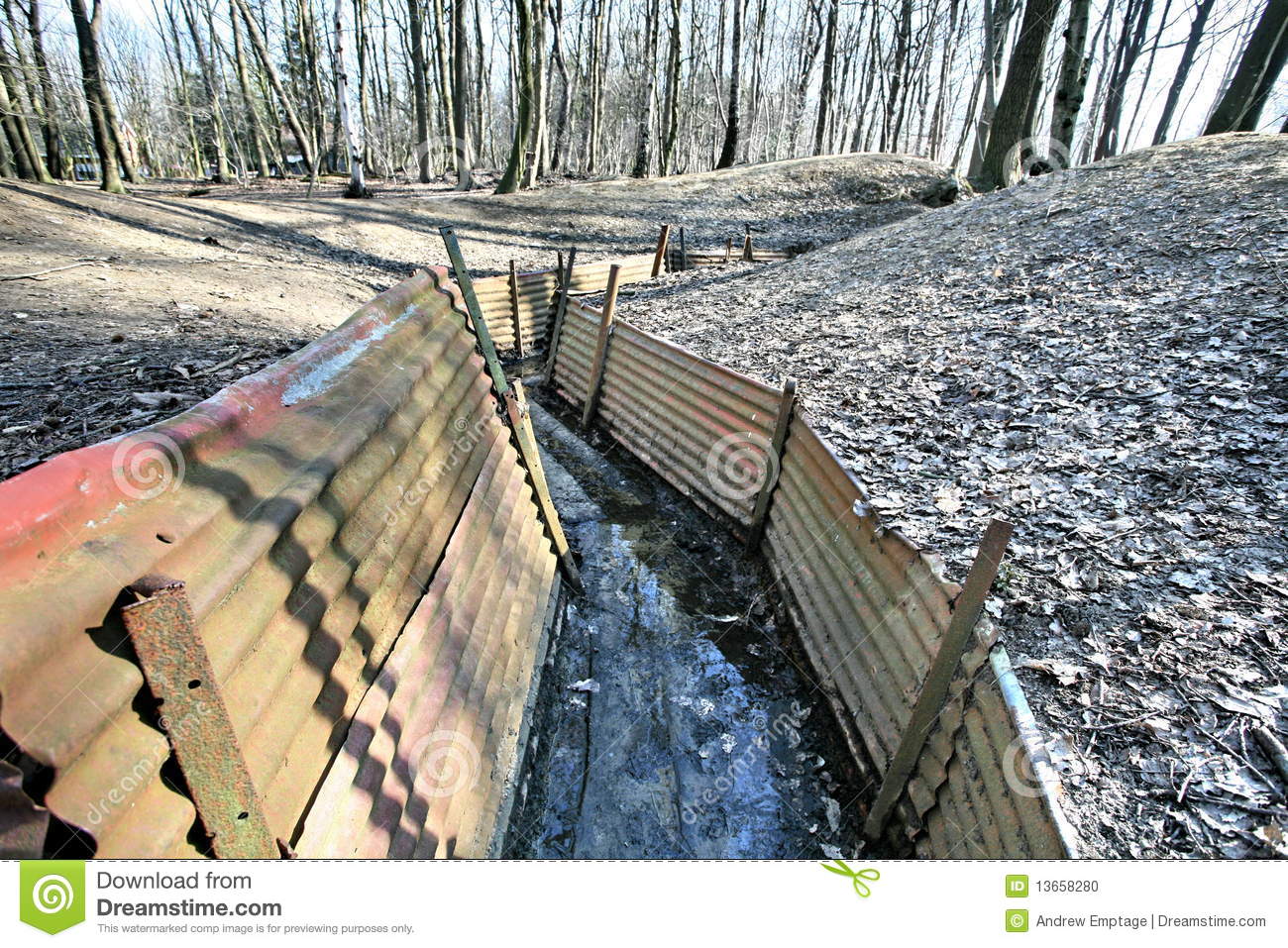In an outdoor scene, tall, leafless trees in the background stand starkly against a mostly cloudy sky, suggesting it's late winter or early spring. The dry ground is strewn with faded, brownish-grey dead leaves, emphasizing the season's end. Down the center, a small pathway winds, directed by a flimsy metal fence that appears to be constructed from corrugated aluminum panels. This mustard-yellowish, tan, and beige fence has angular, horizontal stripes, mimicking roofing material. It guides the pathway as it bends towards the right. The scene is framed by watermarks with swirls from Dreamstime.com, indicating the image is for previewing purposes, with specific credits to Andrew Emptage on the lower right.